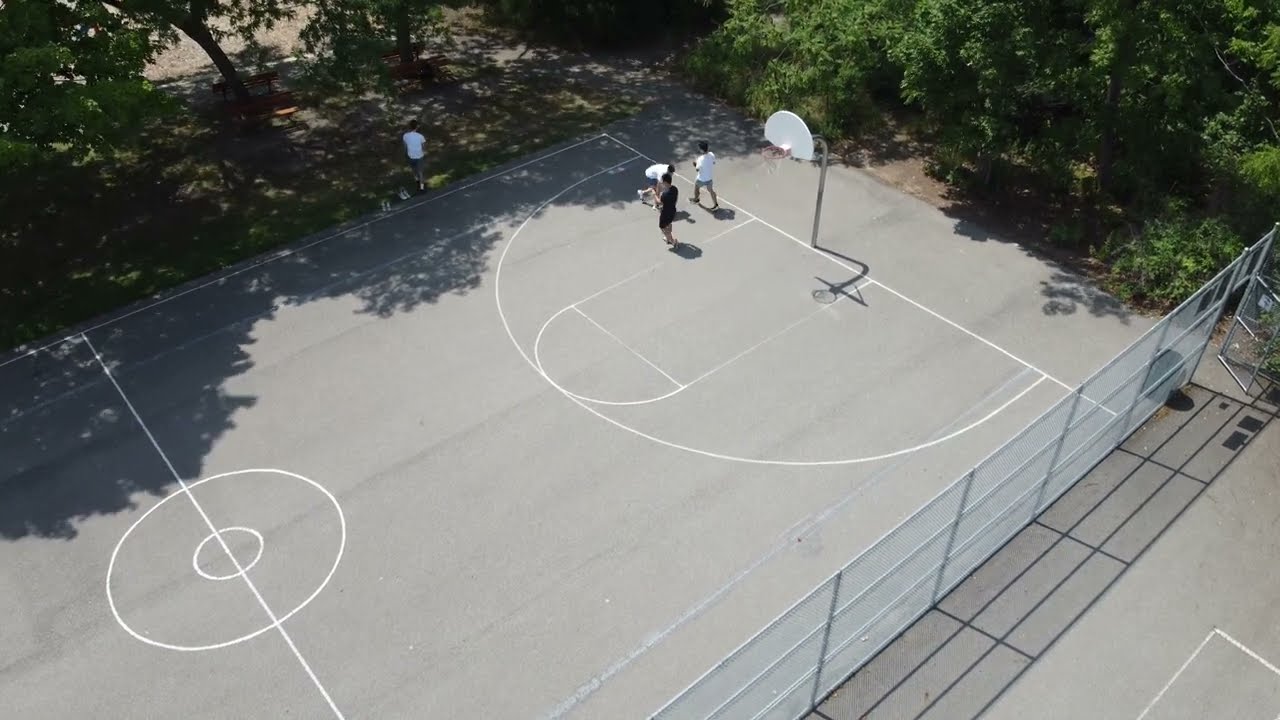This is a detailed aerial photograph, likely taken from a drone, capturing an outdoor basketball court on a gray concrete surface with white lines indicating a well-used playing area, as some of the markings have worn away from frequent activity. A metal chain-link fence runs along the right side of the court, featuring a gate that leads to another area, which appears different—possibly a tennis court or a parking lot, as the markings are not for basketball. The scene is shaded partially by surrounding trees, with dense foliage visible particularly in the upper right corner. There are four young men visible in the image: three actively on the court and one on the sidelines. Three of them are wearing white shirts, and the fourth is in a black shirt. The sun casts shadows from the trees, enhancing the natural setting of this recreational area.